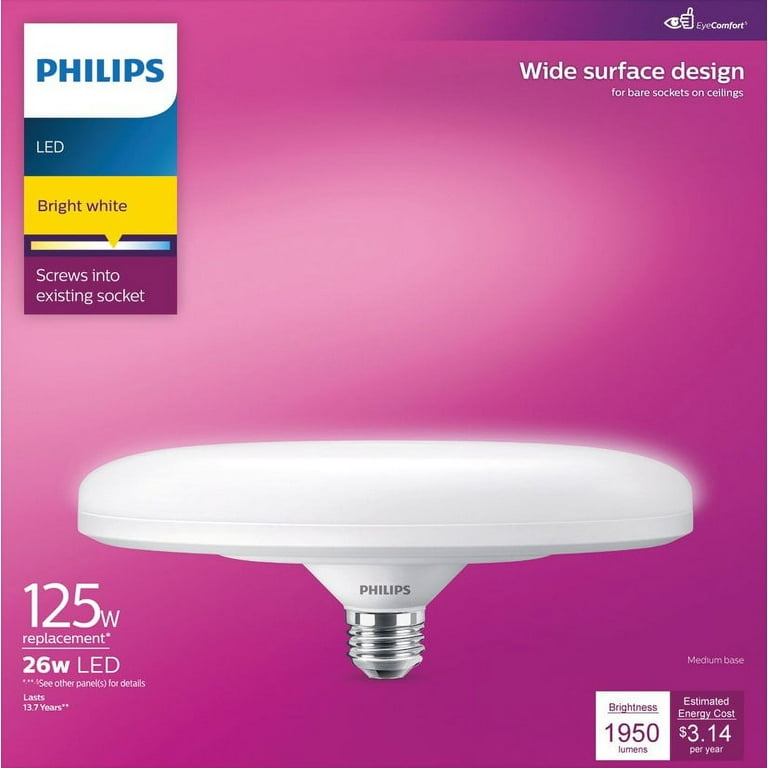The image showcases a box for an unusual Philips LED bulb against a bright pink background that transitions to white at the top. The upper left corner features the Philips logo in blue capital letters on a white rectangular segment, followed by a smaller blue rectangle with white text that reads "LED." Below that, on a yellow background, dark purple text states "Bright White." Further down, another segment in a slightly pinkish-purple declares "Screws into existing socket" in white text. 

In the upper right corner, white text on the pink background says "Wide surface design for bare sockets and ceilings" and "Eye Comfort." The lower half of the box displays an image of the bulb, which is described as a long, flat, and potentially donut-shaped light. The bulb has a conical narrowing element labeled "Philips" with the screw base in silver. The lower left corner of the image contains white text that reads "125W replacement" with an asterisk, followed by "26W LED." 

Additionally, the lower right corner features two white squares; one indicates a brightness of "1950 lumens," while the other states the estimated energy cost of "$3.14 per year." The bulb is expected to last approximately 13.7 years.